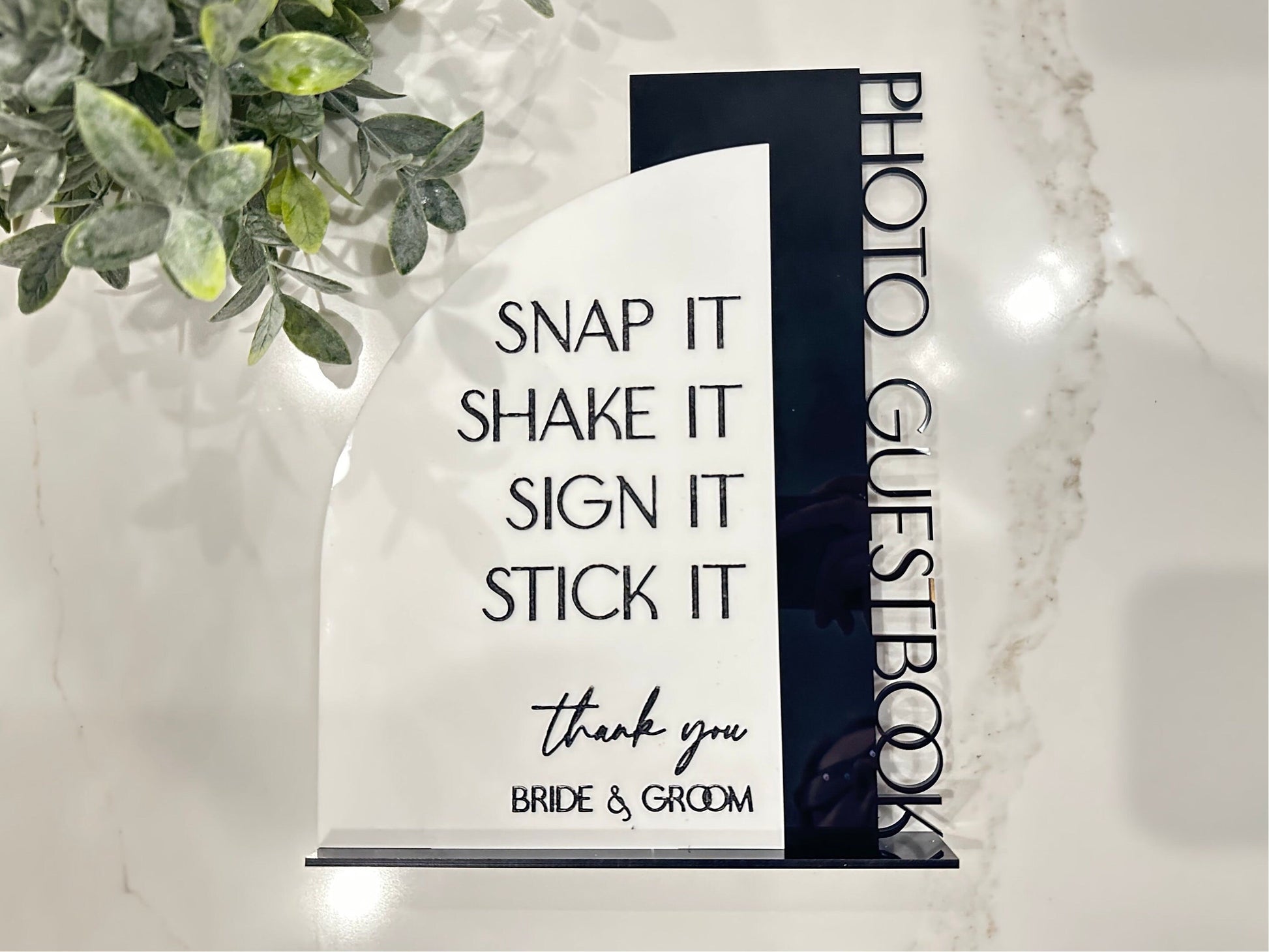The image depicts a wedding guest book display set on a white marble table. In the top left corner, there is a houseplant with visible leaves. Central to the image is a sign with black text reading, "Snap it, shake it, sign it, stick it. Thank you bride and groom." To the right, against a white background wall, a vertical black bar states "Photo Guest Book." The display appears to encourage guests to take photographs and add them to the guest book, adding a personal touch to the bride and groom's wedding keepsake. The arrangement, although not upright as one might expect, lies flat on the table, presenting a charming, interactive element for the wedding.